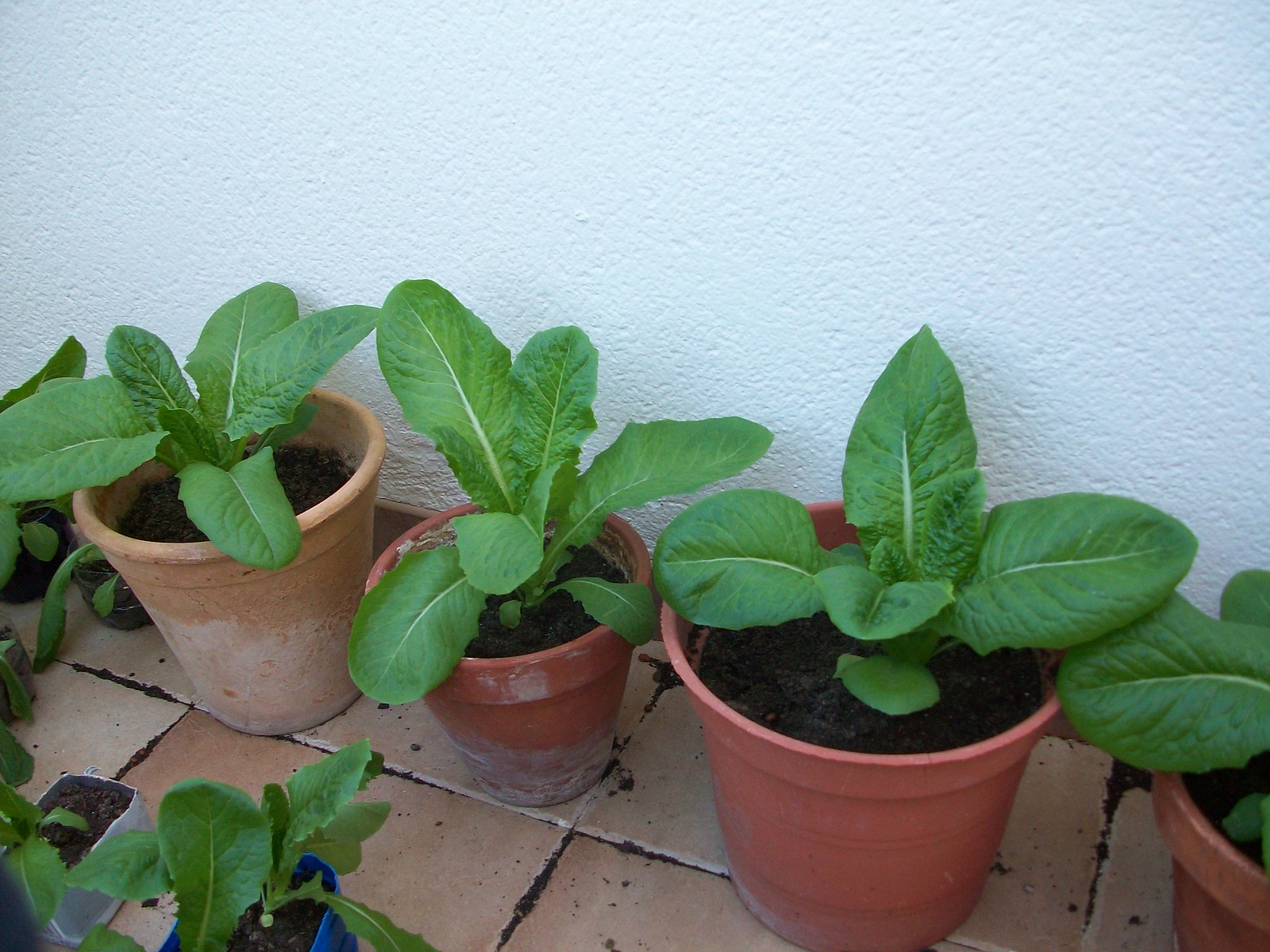The image features an exterior white stucco wall with a collection of terracotta plant pots arranged on paler-than-terracotta red pavers. Most of the containers appear to be actual clay pots, while one might be plastic designed to imitate clay. Each pot houses lush green plants that are likely young lettuce, possibly interspersed with other greens like young Gerbera daisies. To the bottom left, there are additional smaller containers, including makeshift planters repurposed from a blue oval laundry detergent jug and the bottom of a milk jug, also growing young lettuce. This appears to be a quaint container vegetable garden set up next to a house. On the far right, a partially visible fourth pot intrudes into the frame, hinting at more plants beyond the main focus.